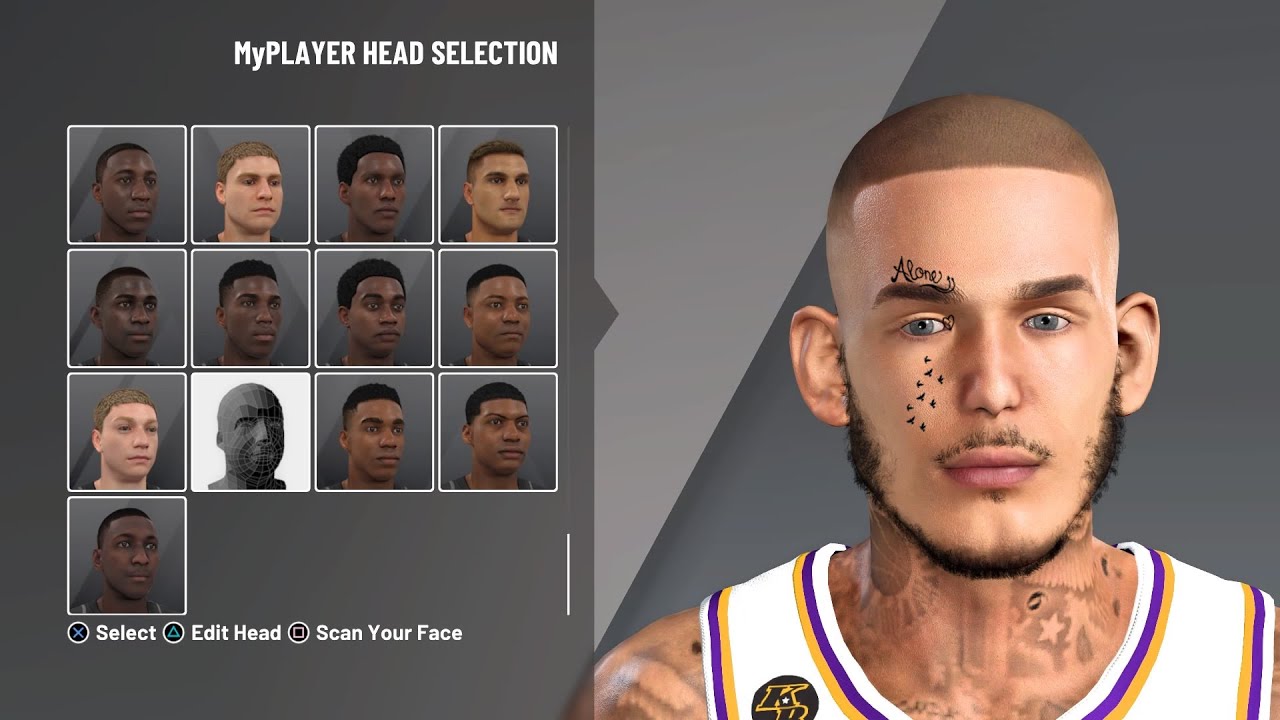**Detailed Caption:**

This image is a screenshot from an NBA video game, featuring the "My Player Head Selection" menu. The background comprises two tones of gray: a darker gray on the left and the right, with a white-gray triangular section in the middle. The title "My Player Head Selection" is prominently displayed at the top in white font, with the top-left corner of the screen specifically highlighting this heading.

Below the title, there are four rows of various character heads, showcasing diverse racial representations, with a noticeable number of heads of African descent. All the heads depicted are male and rendered using computer graphics, each facing towards the right.

At the bottom of the screen, there is an interactive menu corresponding to PlayStation controller commands. It includes options labeled as: "X Select," "Triangle Edit Head," and "Square Scan Your Face."

On the right side of the screen, a selected head is prominently displayed. The chosen character appears to be a mixed-race man in his mid-20s with distinguishing features. He has a shaved head, piercing blue eyes, and multiple tattoos: one on his neck, a tattoo on his cheek, and another above his left eyebrow. His facial hair consists of a mustache and black mutton chops. He is dressed in a white, blue, and orange striped jersey, further adding to his distinct look.